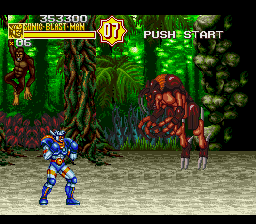The image is a screen capture from an old two-dimensional video game featuring a jungle-themed backdrop. In the bottom left corner stands a humanoid character dressed in a combination of dark blue and light blue attire, accented with touches of orange. The character is unarmed and stationary. To the character's immediate right, there is a menacing, red, demonic monster equipped with large claws and spikes protruding from its feet. A monkey can be seen hanging in the top left portion of the screen, adding to the jungle ambiance. At the top of the image, a health bar labeled "Sonic Blast Man" is visible on the left, while the phrase "Push Start" appears on the right.